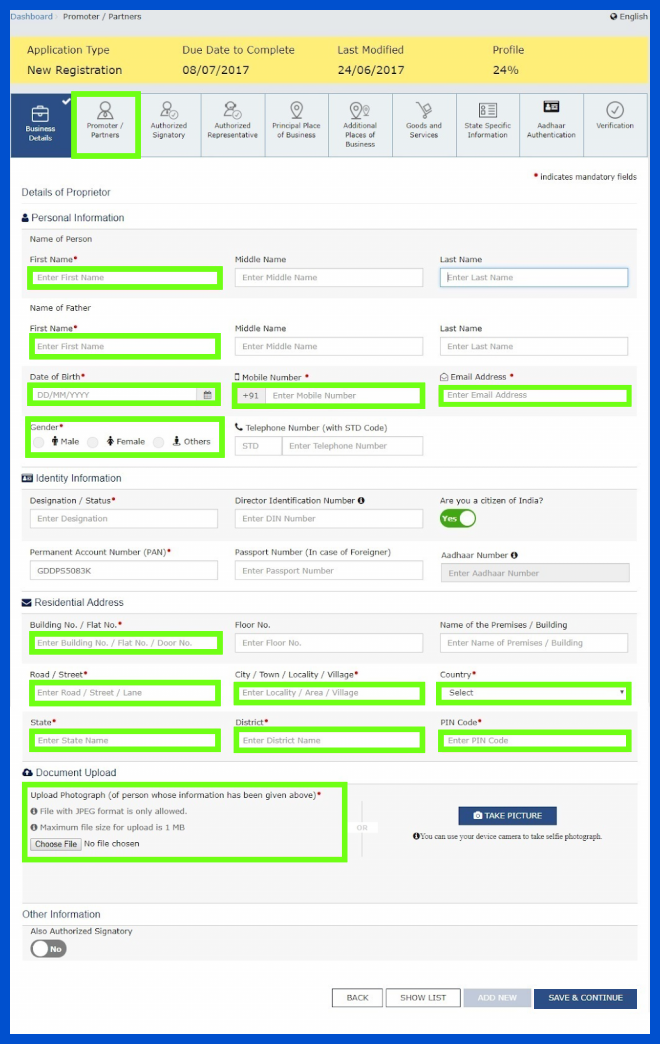**Detailed Caption:**

The image showcases a densely populated web page belonging to "Dashmore Promoter Partners." The page appears pixelated, indicating a poor resolution, but various elements can still be identified.

At the top, a prominent yellow bar details several application specifics:
- **Application Type:** New Registration
- **Due Date:** Complete, with the date 08.07.27.17
- **Last Modified:** 24.06.2017
- **Profile Completion:** 24%

Beneath this header is a menu with various options, including:
- **Business Details**
- **Defaults/Details**
- **Promoter Partners** (highlighted within a lime green square)
- **Authorized Signature**
- **Authorized Representatives**
- **Principal Place of Business**
- **Goods and Services**
- **State-Specific Information**
- **Adhere**
- **Authentication and Verification**

The main form below these options is divided into multiple sections:
1. **Personal Information:**
   - Fields for First Name, Last Name, Date of Birth, Mobile Number, Email Address, and Gender, all surrounded by lime green boxes.
2. **Identity Information:**
   - Contains additional identity details not explicitly listed.
3. **Residential Addresses:**
   - Comprises fields for Building, Road, Street, State, District, Pin Code, Country, and City/Town, also within lime green boxes.
   
At the end of the form, there’s a **Document Upload** section, designated in a lime green box, specifying:
- JPEG format only, maximum size of 1 megabyte
- An option to take a picture directly
  
At the very bottom of the form are buttons for navigation and saving progress:
- **Back**
- **Show List**
- **Add New**
- **Save and Continue**

The overall layout suggests that this web page is an exhaustive fill-in form designed for detailed data collection.